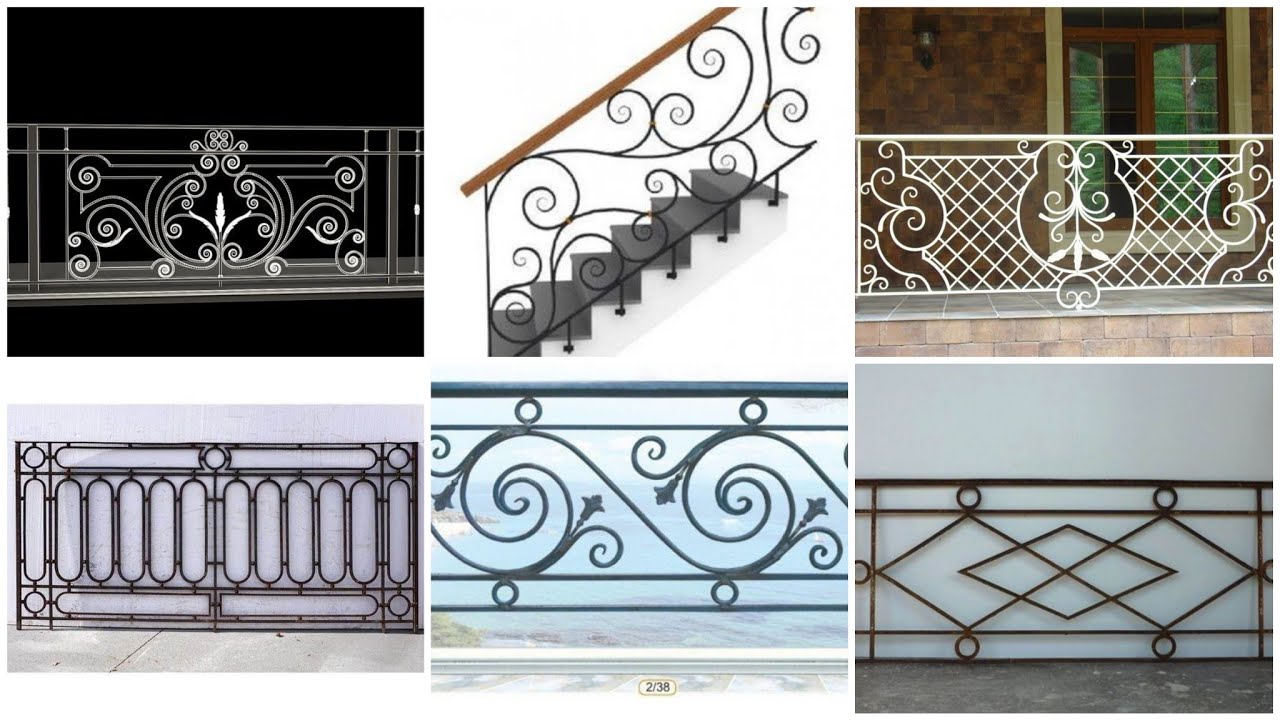The image is a collage of six distinct decorative railings, arranged in two rows of three. Each railing features unique metalwork designs, displaying an array of intricate patterns including swirls, circles, arcs, and interlocking diamonds. The railings vary in color: two are white, two are brown, one is black, and one is gray-blue. One railing, showcasing a glass design with a lot of swirls, appears against a black background. Another, designed with bars and intended for a staircase, features a brown handle and is displayed on a real set of stairs. A third railing, white with swirls and a checkered pattern, is mounted atop bricks. The fourth example is a black railing with oval and circular details laid flat on a white surface. The fifth railing, with intricate swirls and circular details, is set against a blue background. The last railing, brown with circles and diamond shapes, is shown standing upright on a dark gray floor against a white background. Some images depict the railings in realistic settings, while others isolate the designs against plain backdrops.